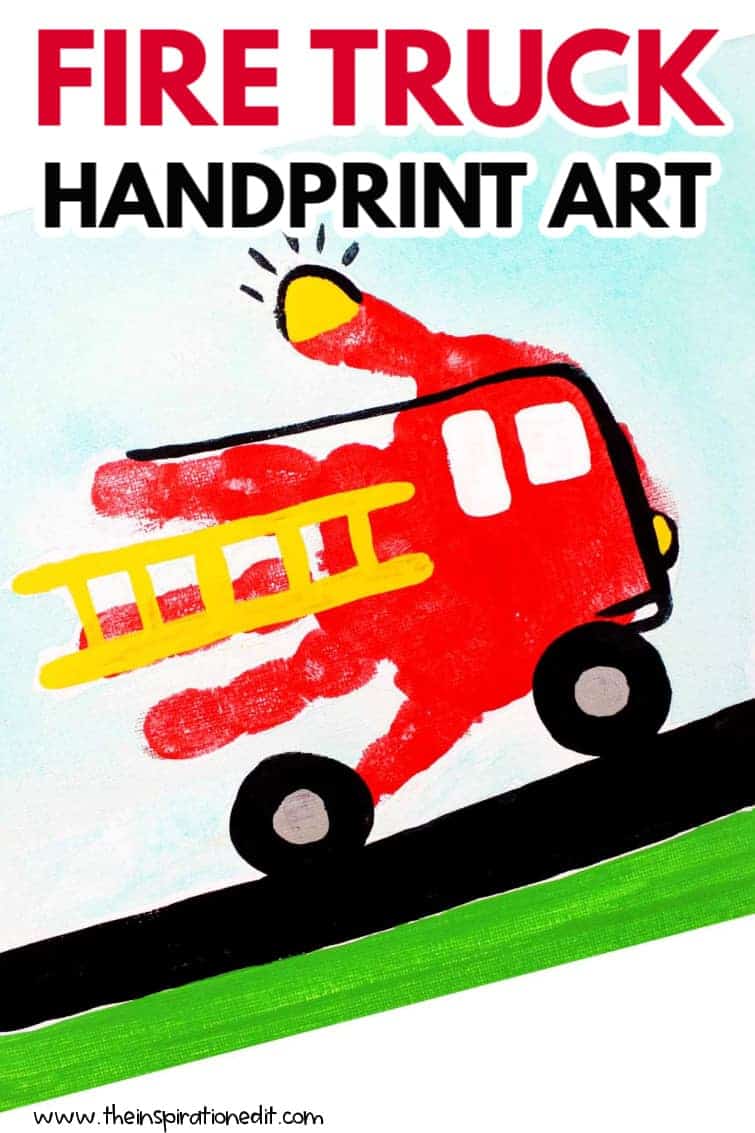This image is prominently featured on the website www.theinspirationedit.com, as indicated by a watermark at the bottom left-hand corner. It appears to be an advertisement or poster for a children’s art project, specifically a "Firetruck Handprint Art" activity. The title "FIRETRUCK" is displayed in bold red capital letters, with the subtitle "Handprint Art" in smaller black capital letters underneath it.

The focal point of the image is a child's handprint, painted red and artistically enhanced to resemble a firetruck. The handprint features two black tires with silver wheels, a white square and rectangle for windows, and a yellow ladder running down the middle finger. The thumb of the handprint has been painted with a yellow tip and outlined in black with small dashes, representing a flashing light. Additionally, there's a semi-circular yellow light at the front of the handprint firetruck.

The background of the poster shows a light blue sky with clouds, a black road that the firetruck is depicted as traveling uphill on, and green grass lining the roadside. This creative and colorful depiction is a perfect example of engaging, kindergarten or preschool-level art activities that parents can do with their children.